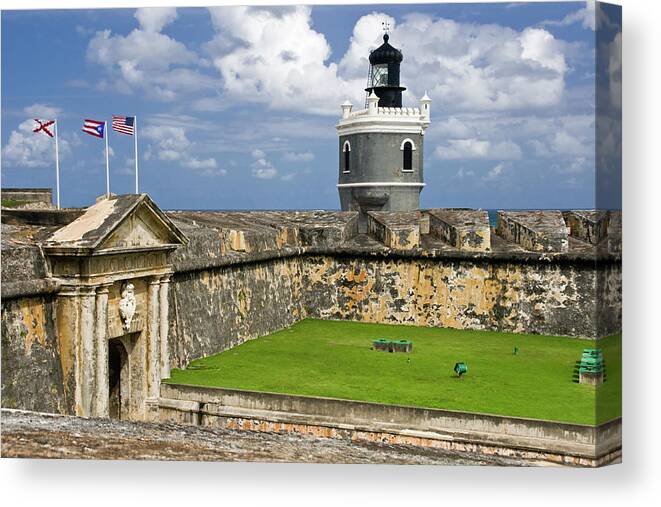The image depicts a canvas print of an old estate that resembles a historical castle, possibly the Alamo in Texas, characterized by its weathered gray stone walls with patches of tan. The canvas, hanging on a white wall, creates a 3D effect noticeable on the right side's shaded dark part. The scene showcases a vibrant green lawn, framed by the aged, crumbling walls. Above the estate, three flags flutter in the breeze: the leftmost flag is white with a red X, the center flag is the Texas state flag with red, white, and blue stripes and a white star, and the rightmost flag is the U.S. flag. A prominent feature in the background is a modern-looking lighthouse, gray with white trim and a black beacon, towering against a backdrop of a blue sky dotted with numerous white clouds.